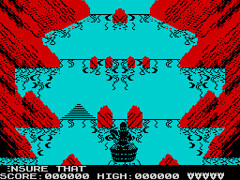The image appears to be a scene from a video game, featuring predominantly red and turquoise colors. On both the left and right sides, there are red rocky structures with vines stretching through the middle, displaying small red elements. The background showcases a turquoise pyramid-like structure, possibly set against a turquoise sky. The foreground includes several rows of black squiggly lines and what seems to be a pyramid at the base, potentially a statue. The bottom of the image features a black border with white text displaying "score: 0000" and "high: 0000," indicating that the game has likely not started yet.